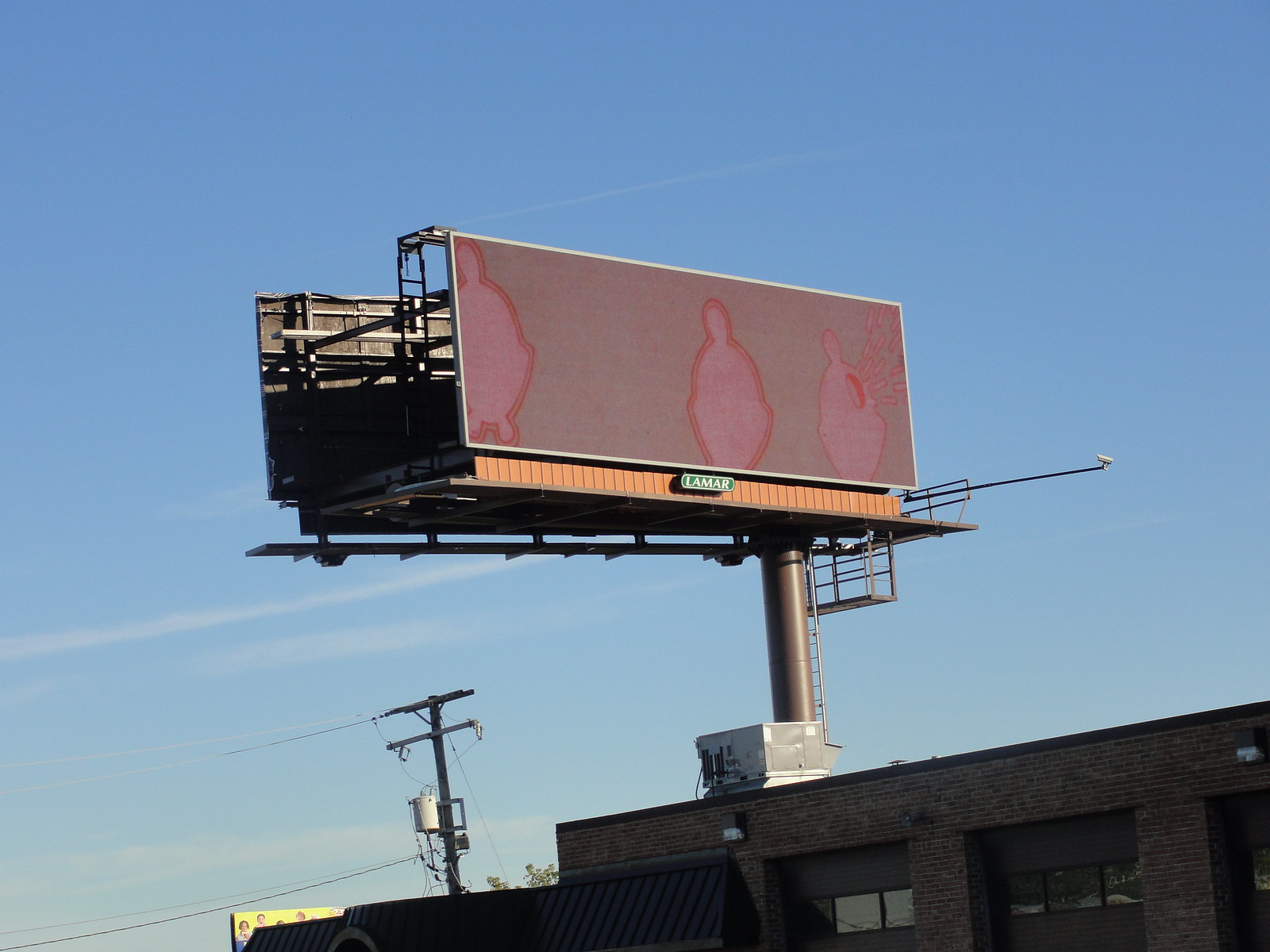This image features a digital billboard situated above a building, angled slightly to the left. The billboard, supported by a single, tall metal pole, is a large rectangle with a paneled base in an orangish-red hue. Below it, a green rectangular logo with white borders and letters reads "Lamar." A surveillance camera mounted on a long metal arm points towards the billboard from its right side.

The billboard itself displays a pixelated, grayish-red background with three heat signature silhouettes of people, presented in round red shapes. The person on the far right has a distinguishable "hole" with an image blurring out from it. The clear, blue sky behind the billboard features faint white trails below the sign, indicative of plane paths.

In the bottom right of the image, the brown brick building supporting the billboard is visible, characterized by a black awning and a gray air conditioner unit on its roof. The building also has garage doors with windows trimmed in black along their tops, and a light fixture installed above these doors. To the left of the billboard, there is a visible telephone pole with overhead wires and another small blue building barely in view. The overall scene is bathed in clear daylight, with only a few scattered clouds in the sky.